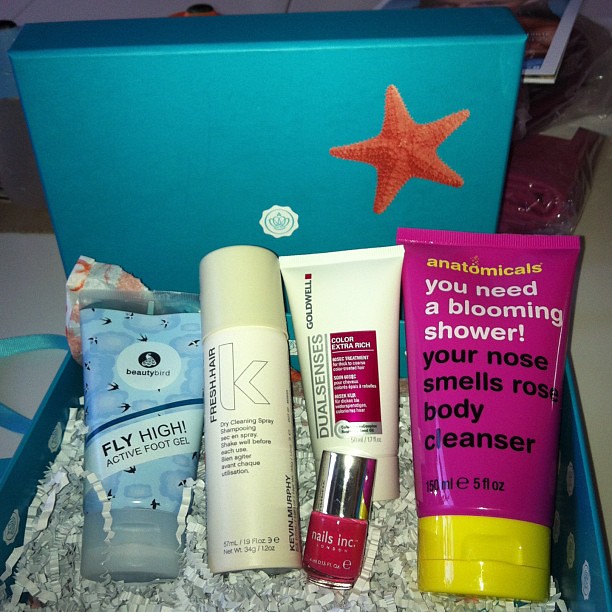This detailed photograph shows an aerial view of a five-inch square blue box filled with shredded newspaper or crinkled paper strips used as padding. The box's lid stands behind it, featuring a plain blue design with a white emblem centered with a blue crown and an orange starfish in the upper right corner.

Inside the box, from left to right, are five beauty items:

1. **Fly-Hi Active Foot Gel** - A blue tube labeled "Beauty Bird Flyhide Active Foot Gel."
2. **Parishum** - A light white colored canister, likely a deodorant, but referred to as "Fresh Air K Dry Cleaning Spray Shampoo" in one description.
3. **Nails Incorporated Red Nail Polish** - A bottle of red nail polish with a silver cap, mentioned as having a gold lid in one description but appears silver.
4. **Color Extra Rich Dual Essence** - A white tube marked "Goldwell Dualness, Color Extra Rich"; further text is unreadable due to glare or distance.
5. **Anatomicals You Need a Blooming Shower Your Nose Smells Rose Body Cleanser** - A large pink tube with a red cap, labeled five fluid ounces.

Additional touches in the image include bits of white and orange paper peeking out from the upper left corner of the box, adding to the colorful, textured arrangement.